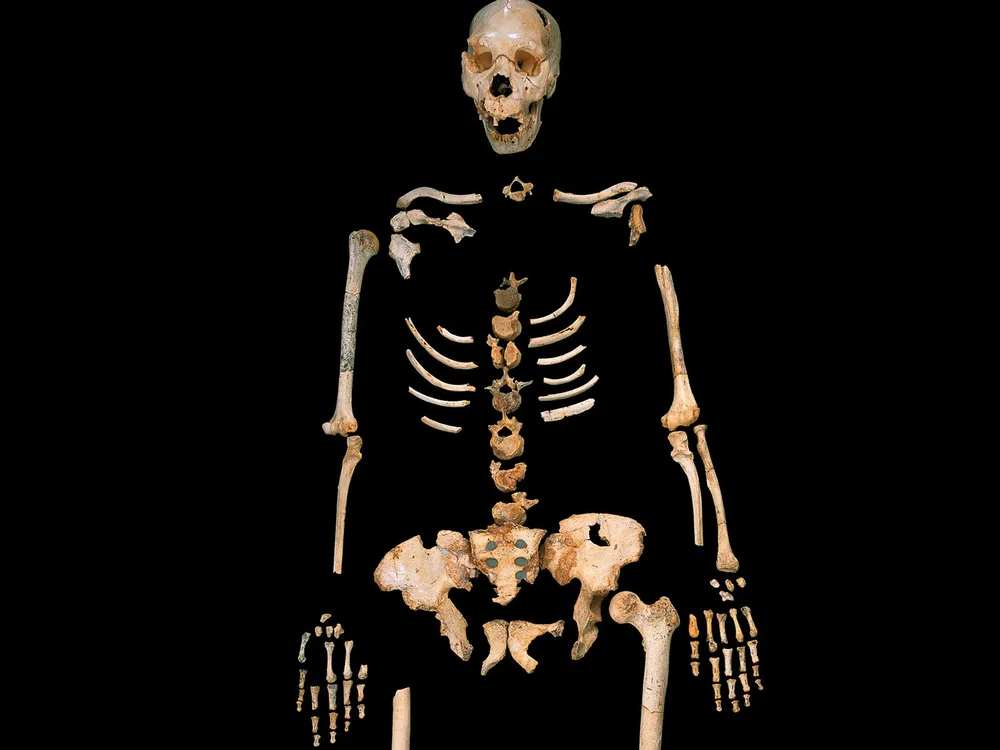The image features a skeleton displayed against a black background, giving it a stark and eerie appearance. The skeleton, which appears to be an ancient and partially decomposed figurine, includes a weathered skull, a collection of ribs, shoulder bones, parts of the spine, and sections of the arm bones. Though incomplete, as several bones such as multiple vertebrae, ribs, wrist bones, and parts of the pelvic area are missing, the arrangement allows viewers to identify key skeletal features. The bones look assembled, suggesting they were recovered and pieced together, yet with an intentional effort to showcase the upper body structure. Despite the missing fragments, the display provides a hauntingly detailed view of an ancient humanoid figure, possibly resembling a Neanderthal or Homo erectus. The dark background amplifies the starkness of the skeleton’s form, highlighting its aged and rugged condition.